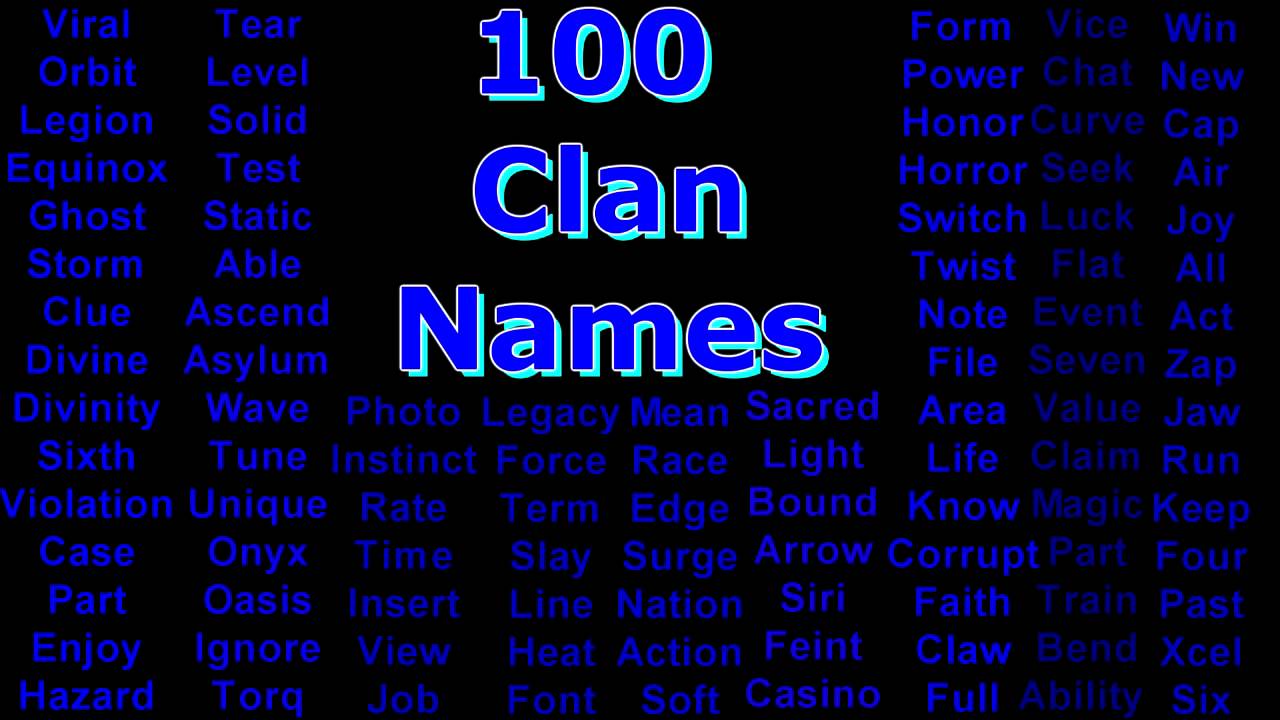The image features a black background with the words "100 Clan Names" prominently displayed in the middle top area. The main text is in a dark blue color with a cyan shadow, creating a visually striking effect. Below the title, the clan names are listed in a medium to dark blue font and are organized in columns to the left, right, and beneath the title. The names are varied and include entries such as Viral, Orbit, Legion, Eponox, Ghost, Storm, Clue, Divine, Divinity, Violation, Sacred, Light, Bound, Arrow, Siri, Faint, Casino, Power, Honor, Horror, Switch, Twist, Note, File, Area, Life, Corrupt, Faith, Claw, Full, Vice, Chad, Curve, Seek, Luck, Fist, Event, Seven, Value, Chain, Magic, Part, Train, Brand, Ability, Excel, Past, Run, Jaws, App, Act, Joy, Air, Cap, Win, and many others. There are approximately 100 clan names in total, presented in no particular order. The stylized text and shadow effect give the image a distinctive, digital appearance.